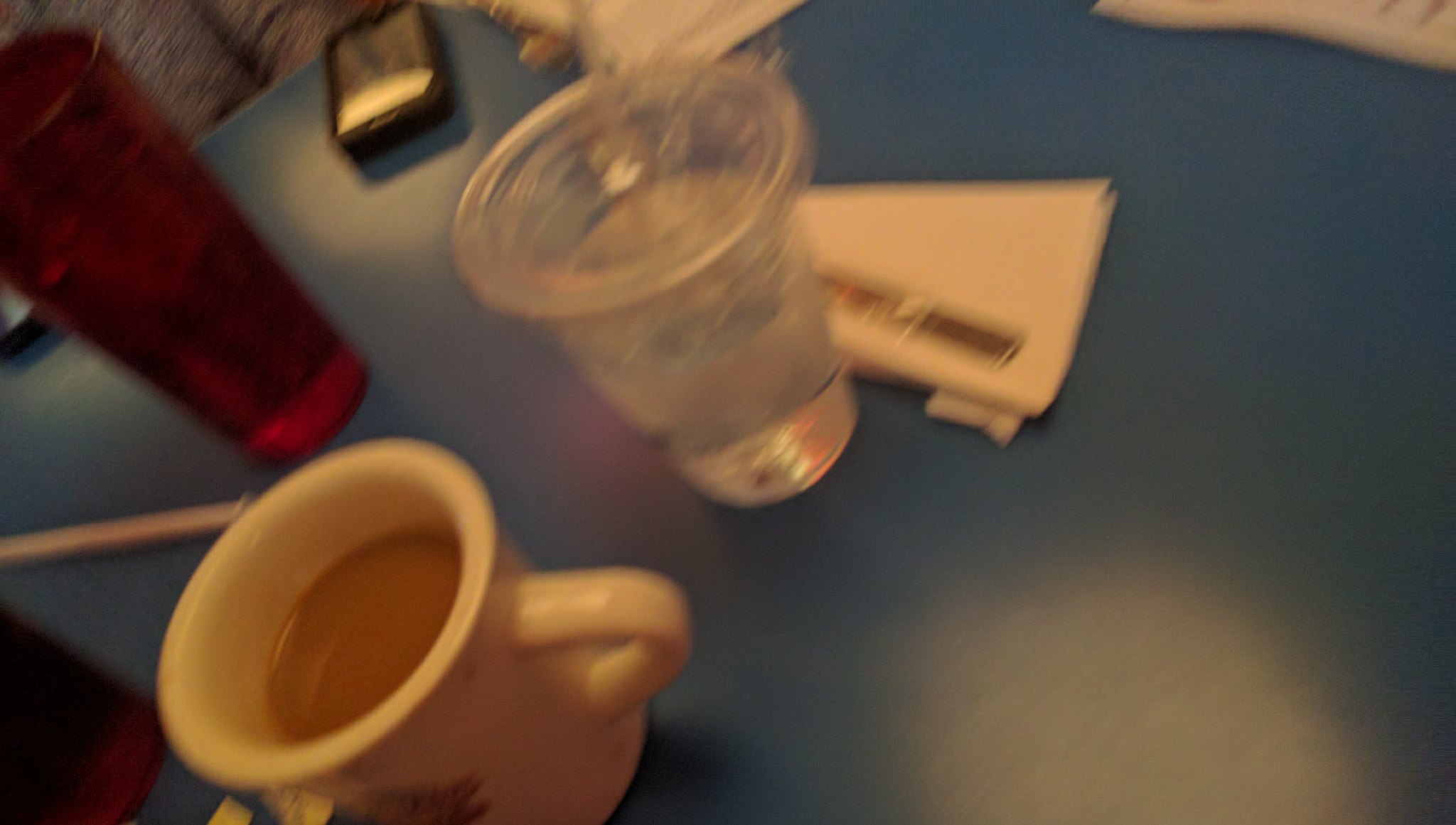The photograph captures a tabletop scene centered around a transparent plastic drinking cup with a plastic lid and a straw, reminiscent of those from fast food restaurants. Behind the cup sits a folded slip of paper. In the bottom left corner of the image, a white coffee mug, filled about two-thirds with cream-laced coffee and bearing an indistinct design, is prominently displayed. Additionally, two large red drinking glasses are visible, adding a splash of color to the composition.